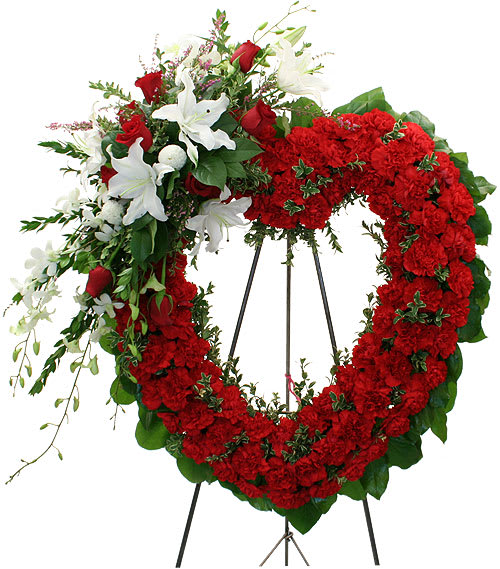The photograph features a heart-shaped wreath crafted predominantly from vibrant red roses set against a stark white background. The wreath, mounted on a black tripod, reveals three partially visible legs extending from its center. The heart's perimeter is densely populated with rows of red roses, interspersed with lush green leaves that add volume and texture. Notable is the top left section of the wreath, adorned with a mixed bouquet of white flowers, additional red roses, and round blossoms, accentuated by delicate small white flowers that drape gracefully over the edges. Within the hollow center of the heart, more green leaves cascade down, adding to the intricate design. The backdrop remains entirely white, focusing attention solely on the intricately decorated floral arrangement and its supporting stand.